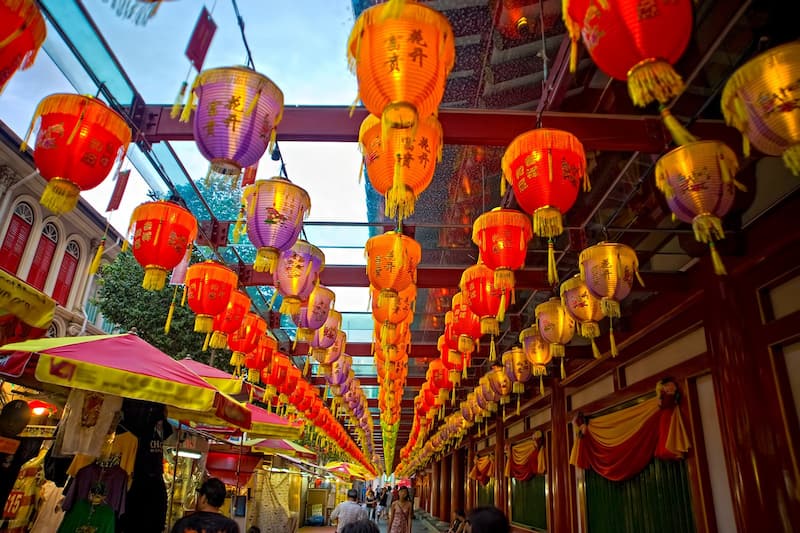This vibrant daytime photograph captures a bustling scene, possibly in Chinatown or a similar Asian district, beneath dozens of oriental paper lanterns organized into colorful rows. Stretching from the foreground into the distance, the lanterns are predominantly red, orange, and purple, each adorned with yellow tassels and marked with Asian script. The lanterns create a lively ceiling above a busy walkway lined with vendor booths selling various items, including t-shirts. The booths are shaded by red and yellow umbrellas. The backdrop is a building with distinctive wooden architecture featuring gold and red drapery over the windows or openings, adding to the rich, vibrant scene. People are seen browsing the booths and walking along the walkway, contributing to the energetic ambiance of the market.